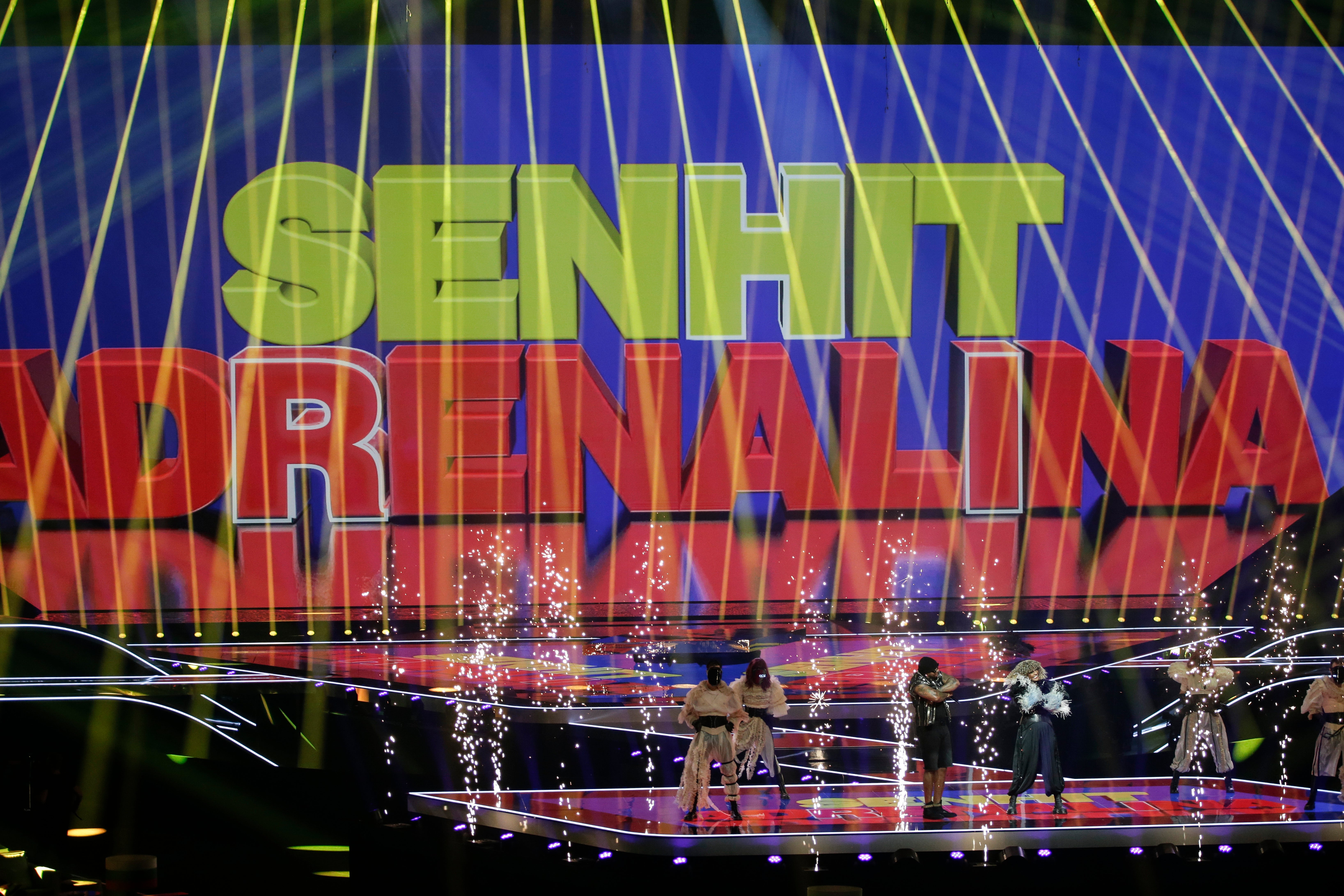The image portrays a dynamic indoor stage performance, featuring six performers. They are standing on a rectangular stage, each adopting a wide-legged stance. Their attire predominantly consists of white robes with black belts, while one performer stands out in large blue pants. The stage itself is illuminated by vibrant pyrotechnics, with sparks shooting into the air. A large screen in the backdrop, set against a blue background, displays the text "SENHIT" in yellow and "ADRENALINA" in red. The performance area is further accentuated by various colored lights, including neon green strobe lights, creating a vividly colorful and energetic atmosphere. The rest of the stage remains black, making the performers and their elaborate costumes stand out even more.